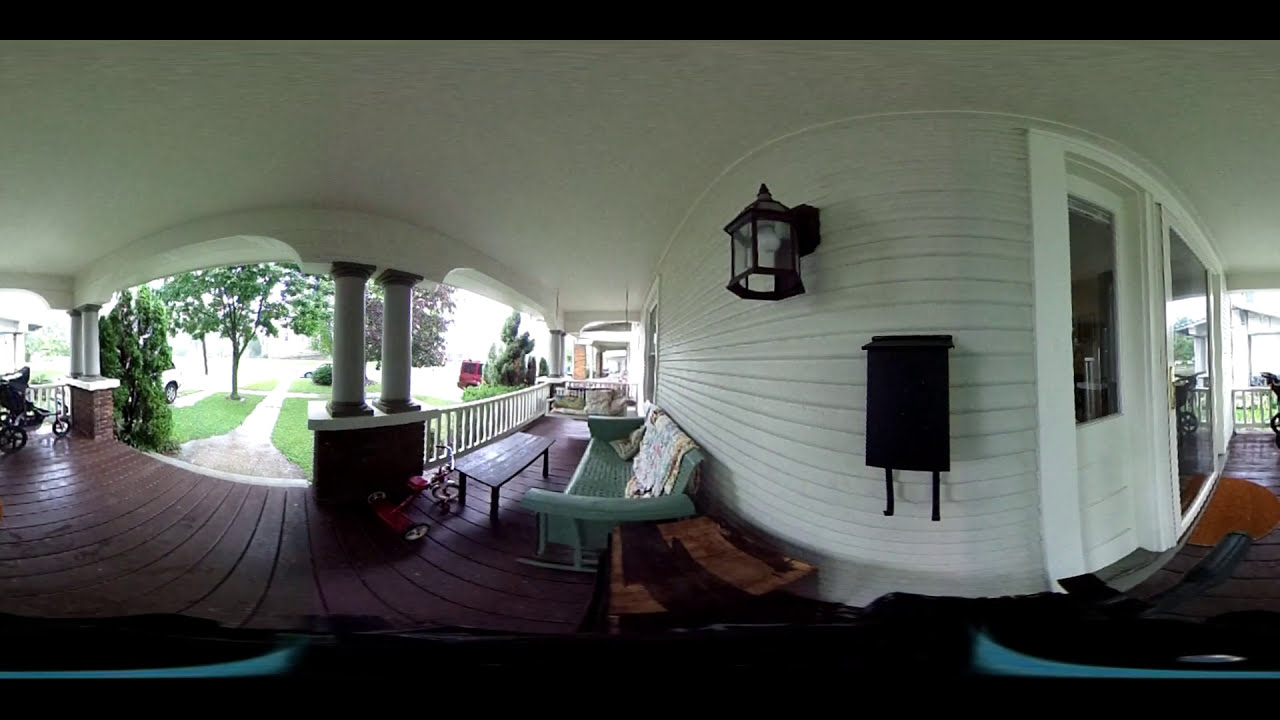This detailed panoramic image captures the front porch of a white house in daylight, presented with a fisheye lens effect that distorts the scene. The porch’s floor consists of dark red wooden planks. White columns supported by brick flank the entrance, and white banisters enclose the porch. A small lawn with trees and bushes surrounds the sidewalk leading to the street, where a parked car is visible.

At the center of the porch, a faded green bench, draped with throws, sits beside a small table. A tricycle is parked next to this setup. Adjacent to the bench, portions of a wheelchair are visible. The porch features a black metal mailbox and a matching black light fixture with a white bulb, both attached to the house's wall. To the right, white doors and large sliding glass windows reveal the house's siding construction of white slats. Additionally, a three-wheeled black baby stroller is positioned at the extreme left of the image. In the background, another house with a similar porch design is partially visible.